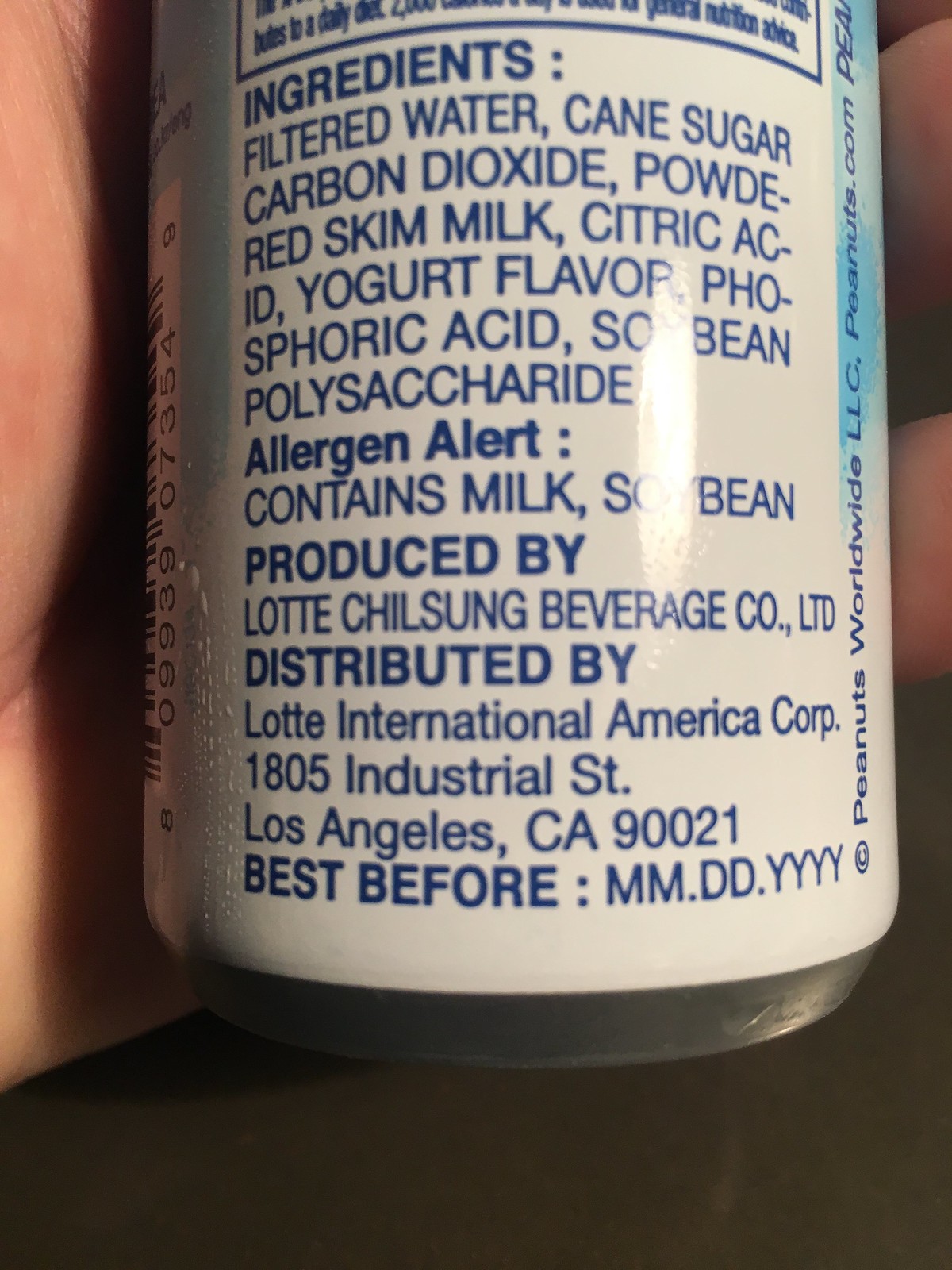The image shows a close-up of a blue and white aluminum can of a beverage, held in someone's hand, with visible condensation on the side. The focus is on the ingredients list written in blue ink on a white background, which details: filtered water, cane sugar, carbon dioxide, powdered skim milk, citric acid, yogurt flavor, phosphoric acid, and soybean polysaccharide. Bolded text underneath the ingredients reads "allergen content: contains milk, soybean." Further details include "produced by Lotte Chilsung Beverage Co. Ltd." and "distributed by Lotte International America Corp., 1805 Industrial Street, Los Angeles, California 90021." The can also features a "best before" date which is indicated as "mm.dd.yyyy," a partial barcode on the left, and "Peanuts Worldwide LLC" alongside "Peanuts.com" positioned vertically to the right.